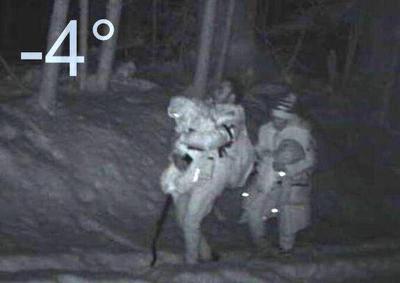This grainy, black and white image, likely captured with a night vision or trail camera, depicts a cold, snowy environment with trees in the background. The temperature, displayed in the upper left-hand corner, reads minus 4 degrees, though it's unclear if this is Celsius or Fahrenheit. Two figures, bundled in very heavy jackets and hats, are walking through the snow-covered landscape. The man in front appears to be holding a walking stick in one hand and carrying a child in the other arm. Following closely behind him, a woman also clad in thick winter clothing, completes the scene. The low image quality and poor visibility contribute to the overall mysterious and harsh atmosphere of the scene.